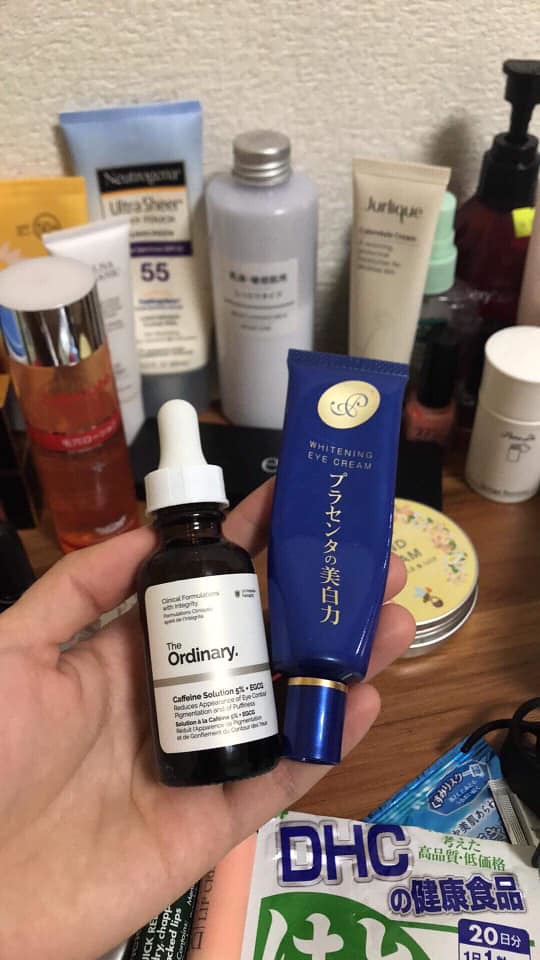The vertical rectangular image features a hand holding two containers. The first container, clasped between the fingers, is a small brown bottle from The Ordinary, labeled with white text and capped with a white dropper lid. The second container, also held in the same hand, is a blue tube adorned with gold-trimmed accents and embossed with a mix of Asian script and English text reading "Whitening Eye Cream." The tube also features a gold logo at the top and a matching gold-trimmed blue lid.

Behind this focal point is a cluttered background showcasing a variety of other bottles, tubes, and containers. Among them is a cylindrical bottle with an orange hue and a silver lid, a white tube with text, a yellow tube with text, a blue and white tube with text, and another cylindrical bottle characterized by a silver cap with a grey appearance. Additionally, there is a brownish tube, a white cylindrical bottle, a very small pot with a tall red lid capped in black, a glass bottle with a green lid featuring a pump dispenser, and multiple little packets and foil wraps. Also visible in the foreground is a flat, cylindrical tray that could potentially hold base powder.

These various beauty and skincare items are all arranged on what appears to be a shelf or a countertop, featuring a rich assortment of colors and shapes that add to the vibrant and dynamic nature of the scene.